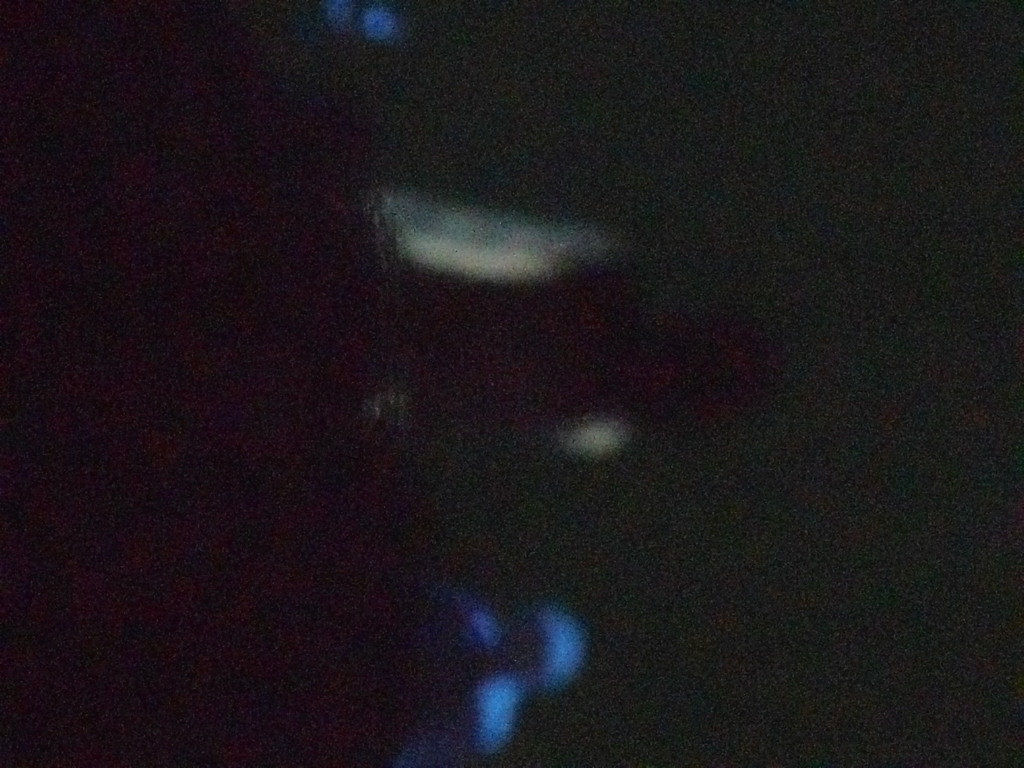This image is an abstract and blurry piece, likely photographed in a low-light setting. Dominated by dark tones, it has a light green tint and exhibits significant noise, making it grainy and blown out. In the center, you can discern the vague outline of a person with dark hair, wearing a black sleeveless shirt. To their right, another figure is faintly visible, bathed in a light blue hue. The foreground features a dark blue mass with some texture atop it, partially obscuring the view. The entire composition includes various shapes and colors, with a distinct elongated blue shape in the lower portion and a yellow blob above it, flanked by two blue squiggles and small blue dots near the top. The combination of these elements gives the impression of an indistinct, possibly digitally rendered or photographed abstract piece.